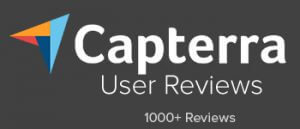The image is a rectangular banner featuring a dark grey background. On the left side, a stylized paper airplane is depicted, angling towards the upper right. The airplane's design transitions from a light blue at the nose to a darker blue towards the center of the wing. The bottom wing shifts from dark blue to red, while the top section of the wing turns orange.

Adjacent to the airplane graphic, the text “Capterra” is displayed in a classic sans-serif font, slightly rounded and white in color. Below this, in a thin, rounded sans-serif font, the words "User Reviews" appear, with both "U" and "R" capitalized. Beneath that, in very small, tightly-spaced white text, it reads "1000+ Reviews," with "R" in "Reviews" capitalized.

The dimensions of the banner are consistent, with the left and right sides matching in height and the top and bottom sides equaling in length. However, the image quality is low, making the text and graphics appear blurry and somewhat fuzzy, particularly noticeable in the "1000+ Reviews" section and around the edges of the paper airplane logo.